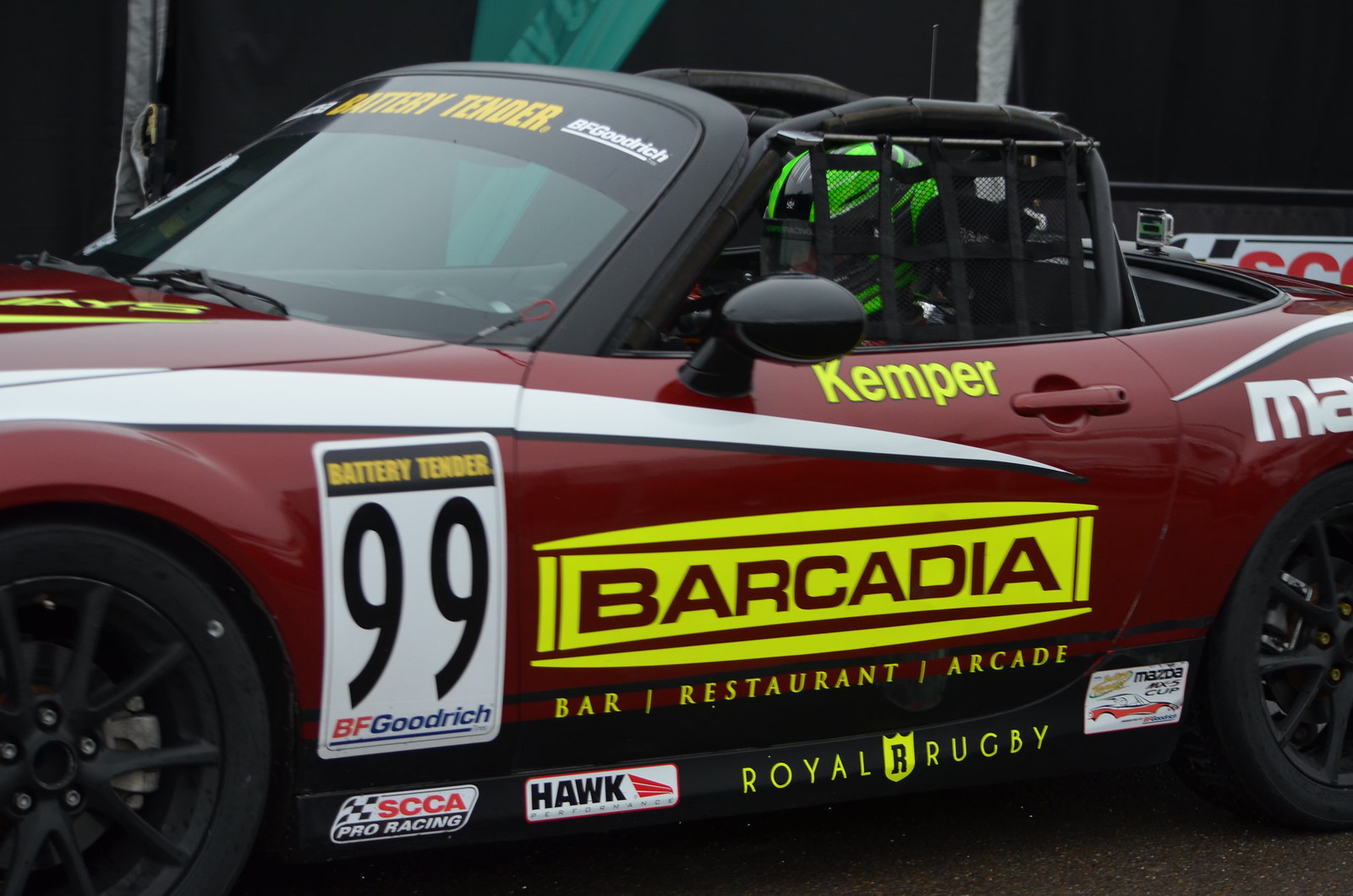In this detailed image, we see a maroon-colored race car centered on an asphalt racetrack, suggesting that it's outdoors and likely taken in the middle of the day. The car, which appears to be a Mazda convertible, is equipped with a black roll cage and is adorned with numerous advertisements and logos. Prominently, there's a white square with the black number 99, indicating its race number. Below this, it reads BF Goodrich. The largest text on the car, in bright yellow, advertises Barcadia Restaurant Bar Arcade. Other notable logos include Battery Tender on the windshield, Hawk, Royal Rugby, Kemper near the door handle, SCAA Pro Racing, and Mazda near the back wheel. The driver is clearly visible, wearing a green and black helmet with a black visor. The overall composition gives a detailed and zoomed-in view of the car, with little of the surrounding background visible.